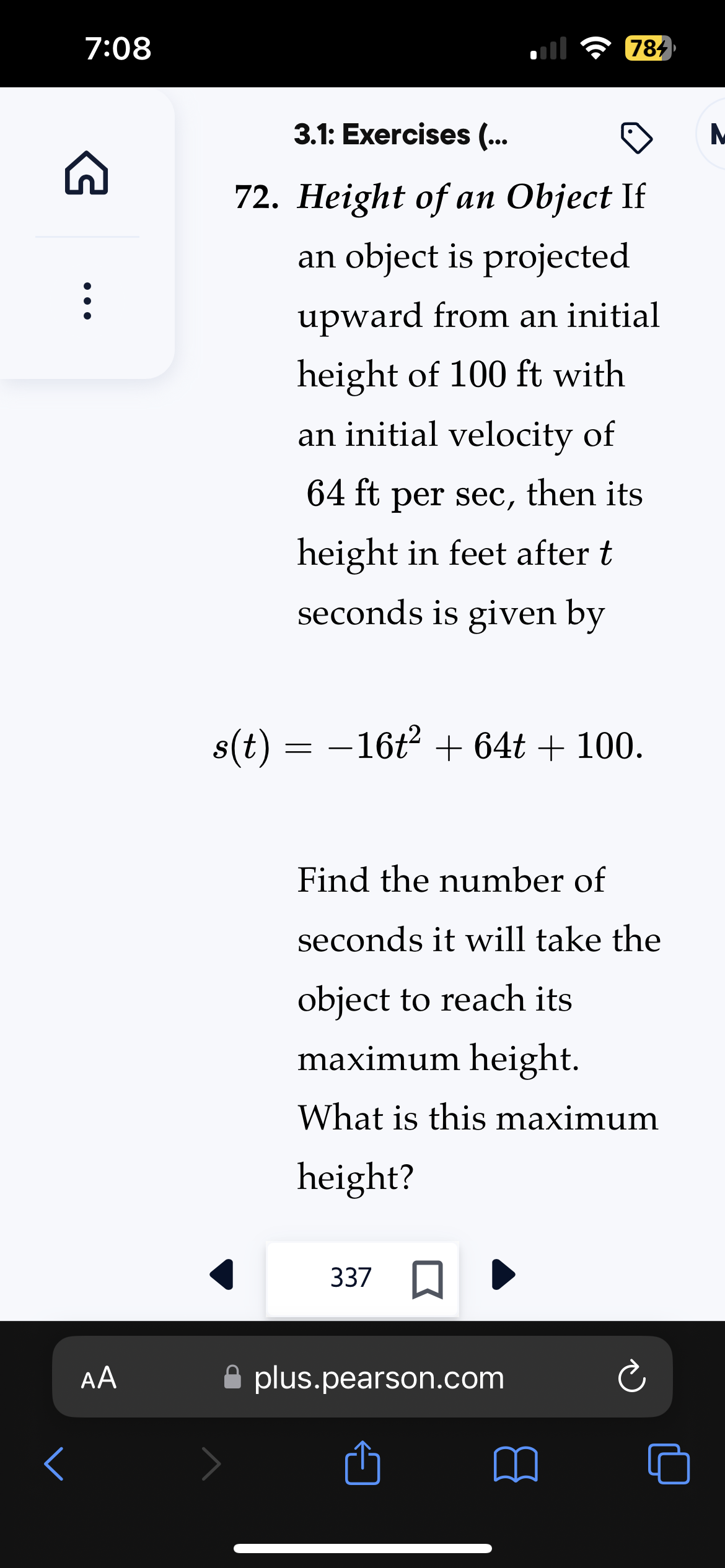In the image, located at the top left corner, the time reads between 7 and 8. On the top right corner, the network signal is depicted with 1 out of 4 bars, accompanied by the WiFi icon and a battery level indicator showing 78% and currently charging. Below these indicators is a mathematical problem describing the height of an object projected upwards. The problem states: "If an object is projected upward from an initial height of 100 feet with an initial velocity of 64 feet per second, its height in feet after t seconds is given by the equation \( s(t) = -16t^2 + 64t + 100 \). Determine the number of seconds it will take for the object to reach its maximum height and calculate this maximum height."